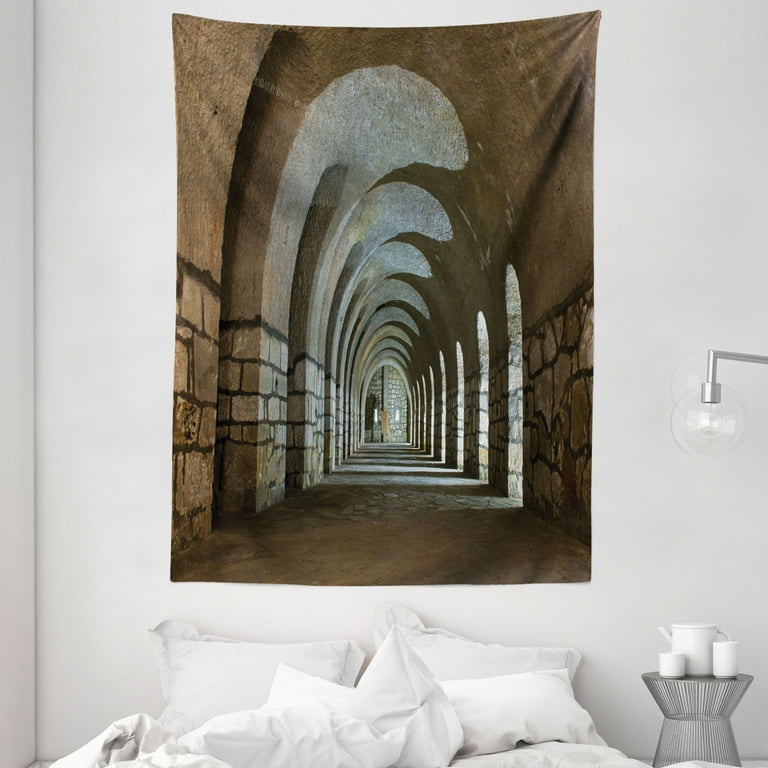The image captures a tastefully decorated bedroom with a prominent tapestry hanging above the bed. The tapestry depicts a long, arched stone hallway reminiscent of a medieval castle, with intricately designed archways on the right that cast curved shadows onto the ceiling and floor. The hallway’s left side is characterized by smooth, tan stone walls, while light pours through the arches, creating a dramatic and atmospheric effect. Below the tapestry, the bed is dressed entirely in white, from the pillows to the duvet cover, exuding a clean and minimalist aesthetic. To the right of the bed stands a sleek, metallic silver nightstand, adorned with a white ceramic pitcher and two matching cups. Above this nightstand, a modern silver lamp with a clear glass globe adds a touch of contemporary design. The entire setup, possibly intended for a catalog or website advertisement, emphasizes the tranquil harmony between the stark white bedding and the rich, historical imagery of the tapestry.